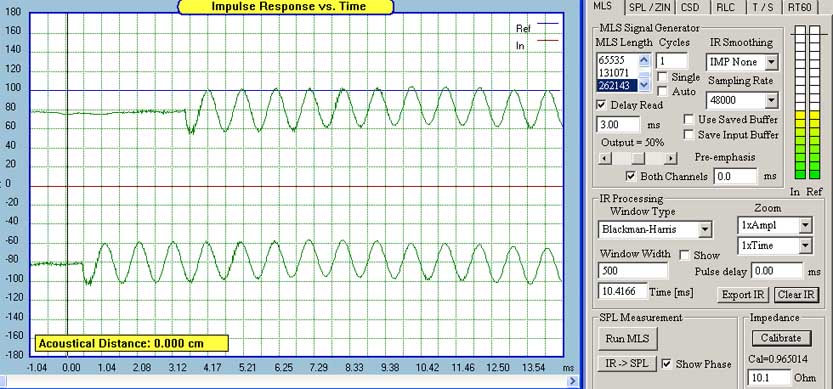The image displays a digitally plotted graph titled "Impulse Response versus Time" with a yellow highlighted background. The graph, framed by a blue border, features two key lines: a blue "REF" line and a red "IN" line, identified in a key at the top right. On the left vertical axis, values range from -180 to 180, while the horizontal axis spans from -1.04 to 13.54 milliseconds. The top line begins at 80, fluctuating in a zigzag pattern up to 100 and down to 60, while the bottom line starts at -80 and oscillates between -60 and -100. At the bottom left, there is a yellow box stating "acoustical distance 0.000 cm." On the right side, a gray panel displays multiple tabs including MLS, SPL, ZIM, CSD, RLC, TS, and RT60, with numerous options such as MLS signal generator, MLS length, cycles, IR smoothing, sampling rate, delay, reuse, save buffer, output, and pre-emphasis. The right side also features a meter transitioning from white to yellow to green, labeled IR processing and SPL measurement, containing various numbers and words.